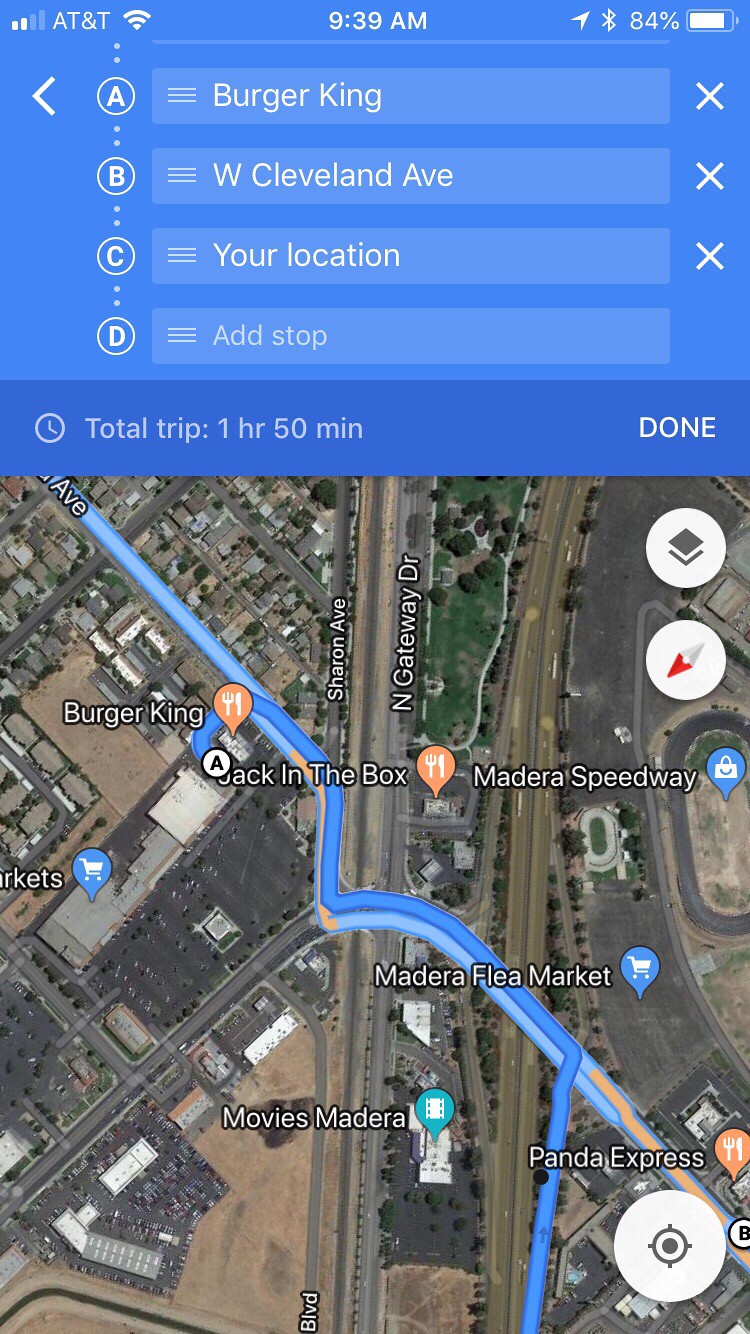This is a detailed screenshot from a mobile device, displaying a mapping application that shows a planned trip with multiple stops. The journey starts at point A, Burger King, and proceeds to point B, West Cleveland Avenue, with point C labeled as "your location." An option exists to add another stop at point D. The estimated total trip time is one hour and 50 minutes, likely assuming walking as the mode of transport. The map is in satellite view and highlights several landmarks, including a Jack in the Box, Madera Speedway, Madera Flea Market, Movies Madera, and a Panda Express, all situated along North Gateway Drive in Madera. Additional details from the device show it is on the AT&T network, the battery is charged to 84 percent, and the time displayed is 9:39 a.m.